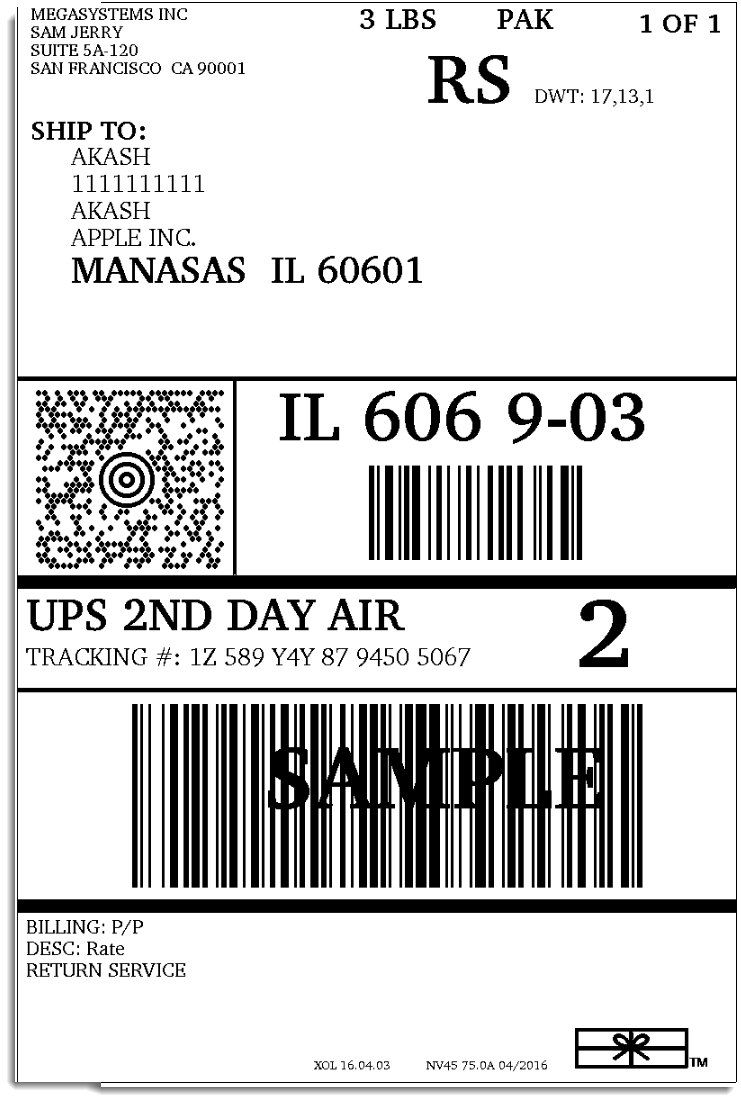This is an image of a detailed, black and white UPS shipping label for a package sent via UPS Second Day Air. The upper left corner features the sender's information, which reads: "Megasystems Inc., Sam Jerry, Suite 5A-120, San Francisco, California, 9001." Directly below, the recipient's details are listed as: "Ship to Akash 111111111, Akash, Apple Inc., Manassas, Illinois, 60601." The label specifies the package weight as 3 pounds and indicates "Pack 1 of 1" along with the dimensions or additional shipping details: "RSDWT: 17, 13, 1." In the middle section, there are both a 2D barcode and a standard barcode, labeled with "IL-6069-03." The service level is marked as "UPS Second Day Air," and the tracking number is prominently displayed as "1Z589Y4Y8794505067." A large number "2" is printed below the service level. Towards the bottom, there is another barcode overlaid with the word "Sample." The bottom section of the label includes various details such as "Billing: P/P," "Description: Rate," "Return Service," and several other numbers and trademarked images including a small illustration of a gift-wrapped box with a bow. The very bottom right corner mentions specific codes and information, potentially metadata for the shipping process: "XOL 160403 NV 45750 A 04/2016."